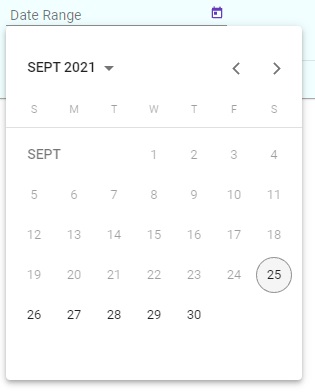This color screenshot, captured in portrait format, displays a detailed view of the calendar feature on a laptop, specifically focusing on September 2021. The current date at the time of the screenshot is highlighted as September 25, 2021, distinguished by a circle around it. The days preceding the 25th are shaded in a lighter gray, indicating that they are no longer selectable, while the days following the 25th—namely the 26th, 27th, 28th, 29th, and 30th—remain clickable. Navigation arrows located at the top right of the screen allow users to move back to August 2021 or forward to October 2021 and beyond. The calendar is set against a clean white background with black text. The header area, slightly shaded, prominently displays the date range, guiding the user through the monthly view.